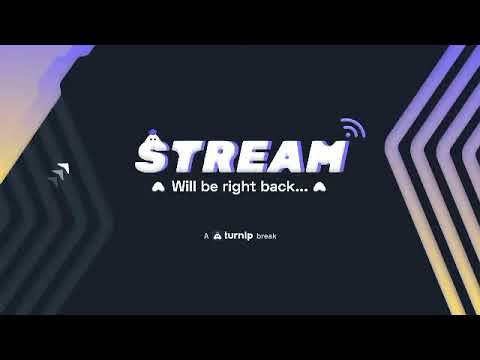The image features a predominantly black background with a light purple, blue, and yellow triangular area in the top left corner. This visually dynamic area contrasts sharply with the otherwise dark backdrop, accentuated by black borders at both the top and bottom. The center of the image prominently displays the word "Stream" in white text, where the letter 'S' has a ghost head above it, and the letter 'M' is topped with a Wi-Fi symbol. Directly below, the text "We'll be right back" is also printed in white, with three dots forming an ellipsis at the end. At the bottom, the words "a turnip break" appear, flanked by three curved lines above the letter 'M', suggesting a playful or whimsical design element. On the right side of the image, there are arrow shapes pointing towards the center, which grow more prominent and purple as they approach the middle, resembling sound waves. The left side features thinner, less defined arrows. The overall image appears to be designed as a screen or slide that someone might use during a streaming break, signaling to viewers to be patient.